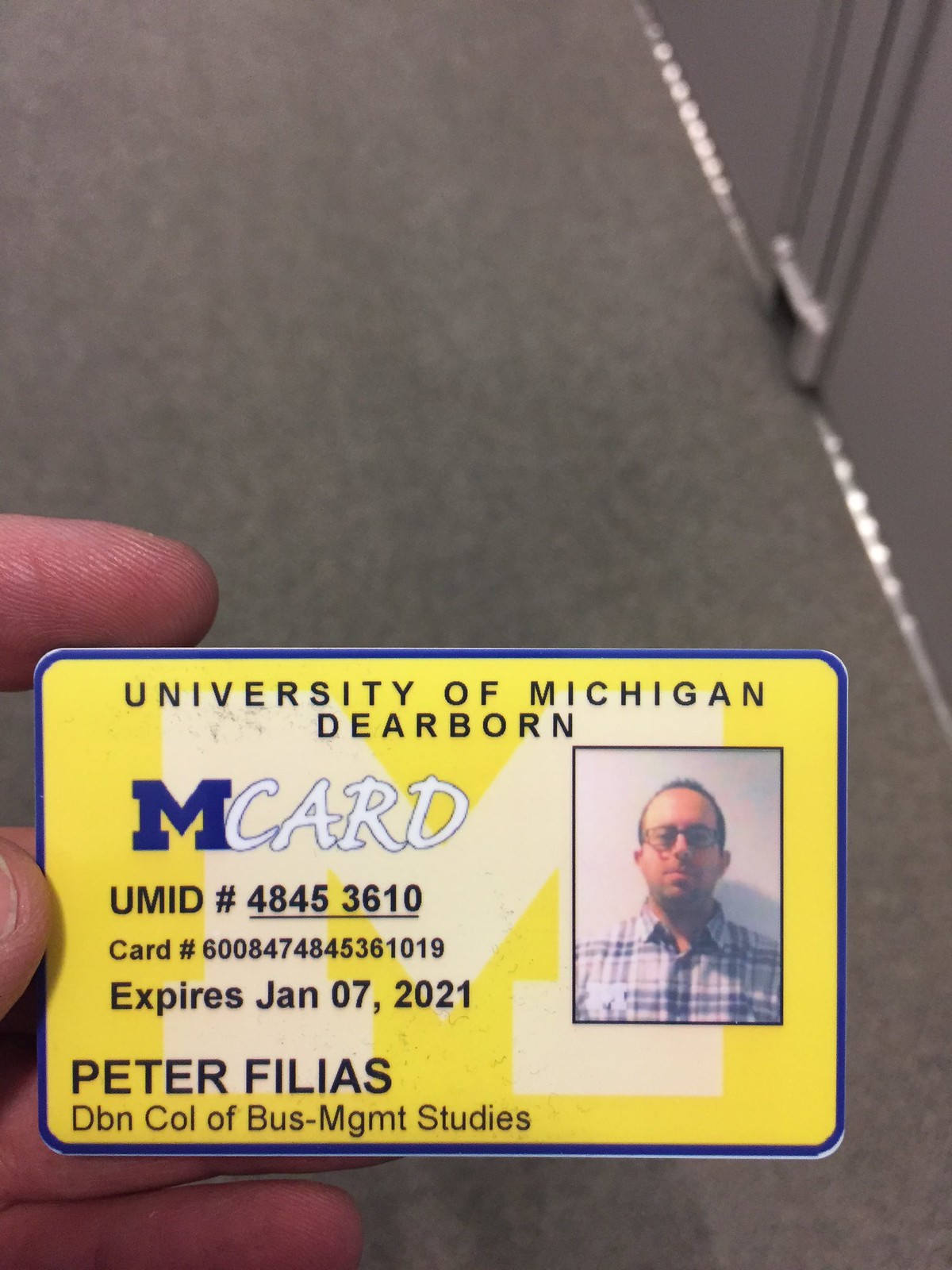A close-up photo shows a hand holding a University of Michigan-Dearborn ID card in front of the camera. The card, which has a blue outline and rounded edges, features a yellow background with a large white capital 'M' subtly printed in the center. At the top, the card states "University of Michigan-Dearborn" in bold black text. Below, it reads "M card," with the 'M' in blue and 'card' in white. Further down, the card displays "UMID, #48453610," followed by "Card, #6008474845361019," and an expiration date of "Expires Jan 07, 2021." The bottom left corner of the card includes the name "Peter Fillius, DBN, Col. of Bus MGMT Studies" in blue text. Additionally, there is a small portrait photo of a man with short dark hair, wearing glasses and a patterned white and blue shirt, likely Peter Fillius himself. The background of the image is slightly blurred, showing a gray carpeted floor and a wall on the top right.